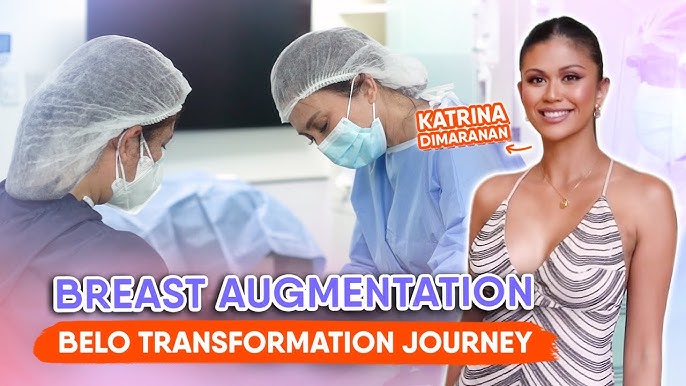This social media graphic is a long rectangular advertisement, split into two distinct images. On the left side, two surgeons are depicted in an operating room, wearing blue paper gowns, medical masks, and hair nets. They are focused on their work, staring intently downward. On the right side, a woman named Kat Katrina Damaranan is shown smiling brightly. She is dressed in a black and white low-cut dress, with her hair pulled back, showcasing her earrings and necklace. Her name is prominently displayed with an arrow pointing to her. Below the images, "Breast Augmentation" is written in bold blue letters, and beneath it, a red banner highlights "Bellow Transformation Journey." The overall design incorporates a colorful gradient and vivid colors, capturing attention and directing viewers to the transformation journey featured.